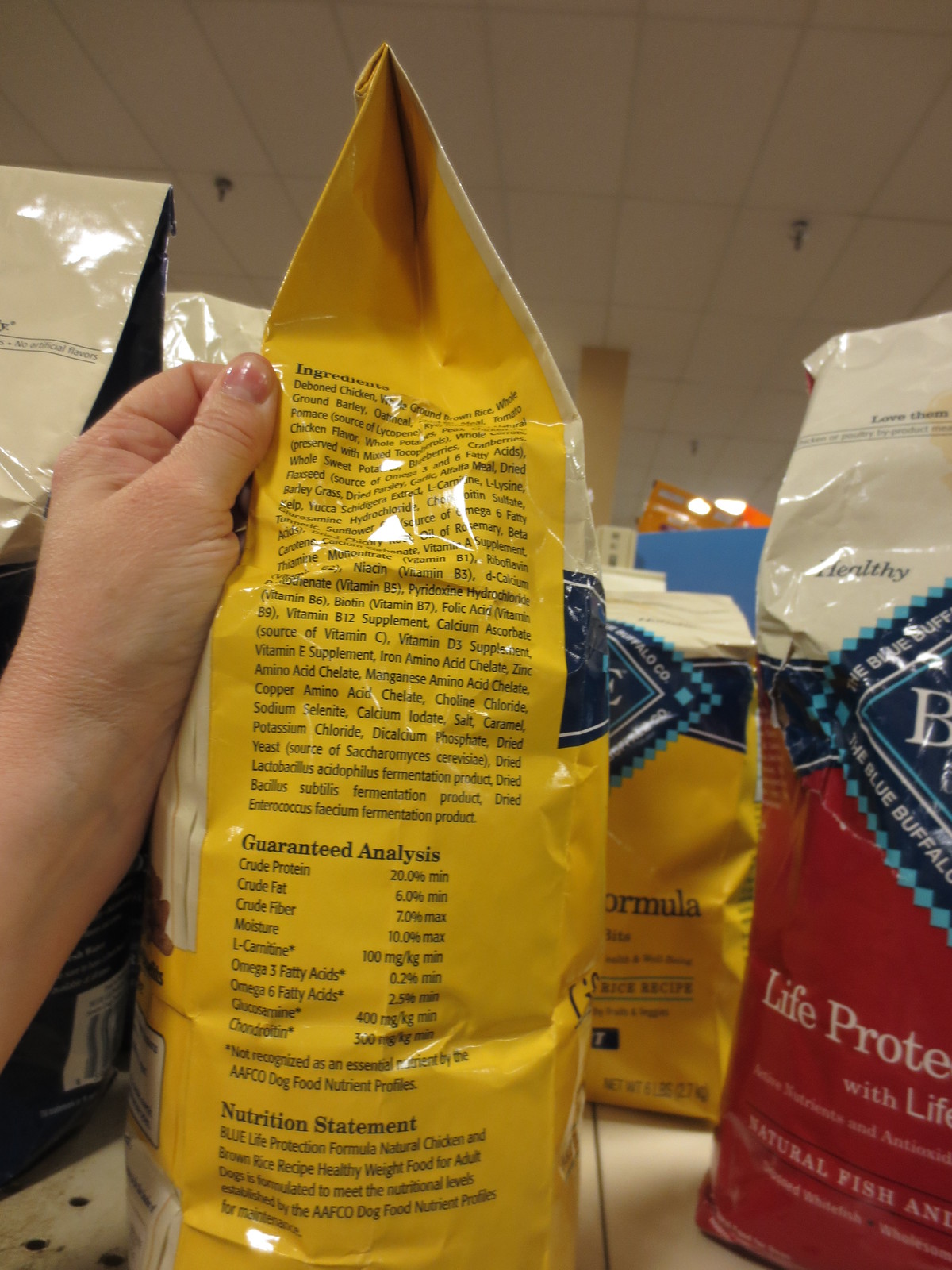In the image, a person's hand, partially extending from the left edge, grasps a yellow-sided bag of dog food by the corner. Surrounding this bag on the display shelf are various other dog food packages, suggesting a store setting. Prominent among the neighboring bags is one on the right, which is white at the top and red at the bottom. This bag features intricate details such as a blue logo encircled by light blue, dark blue, and white edging. A notable letter "B" from the logo stands out, and the text "Life Protect" is visible towards the bottom of the bag. The yellow-sided bag in the center of the image is turned sideways, revealing detailed text including an ingredients list, a guaranteed analysis, and a nutritional statement.